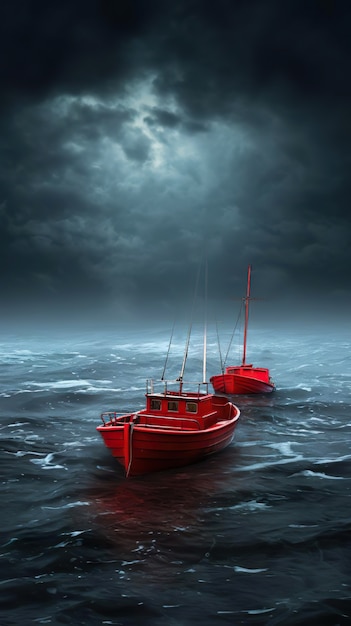This computer-generated, portrait-mode image depicts two vividly bright red boats, reminiscent of tugboats but more akin to sailboats without any visible sails. They sail close to one another, almost like ducks in a row, a boat-length apart on a stormy, choppy sea. The sea is very dark, with almost black waves tipped in white, and the sky mirrors this tumultuous scene with pitch-black clouds. A hidden moon behind the clouds illuminates a small circular area, casting a dim glow. The background transitions from the black stormy sky in the top corners to a slightly illuminated area where remnants of sunlight peek through thick clouds, with this light descending diagonally from the upper left to the center-right. The front boat features three small windows on what appears to be a square captain's cabin, while the boat behind is distinguished by its vivid red mast. The entire scene is devoid of any signatures, trademarks, or text, focusing solely on the dramatic and almost eerie marine landscape with no visible human presence.